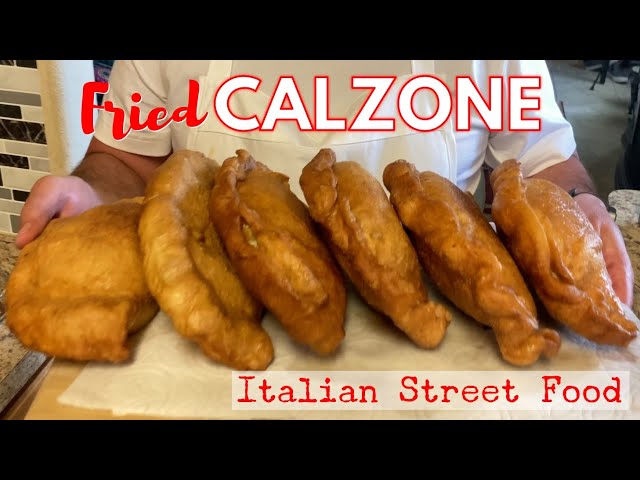In this image, a man in a white t-shirt and apron, with his chest and arms visible, is carrying a tray of six deep-fried calzones. The calzones are light golden brown and appear freshly made. The tray has a piece of paper under the calzones, and above them, a sign reads "fried" in red text followed by "calzone" in white. Below this, in red text, it says "Italian street food." The sign is bordered in black, emphasizing the advertisement for this culinary offering likely from a restaurant or street food vendor. The overall presentation suggests that these calzones are homemade, possibly stuffed with cheese and other fillings.